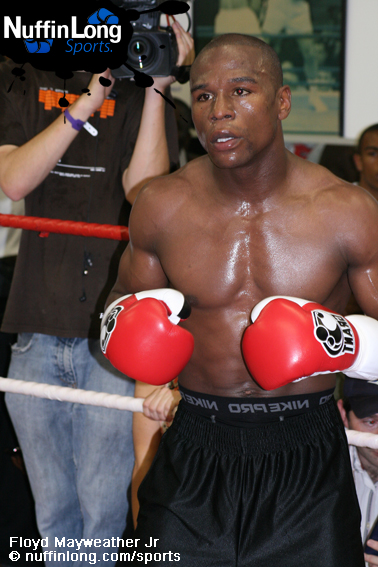This tall rectangular photograph captures a moment in the boxing ring with Floyd Mayweather Jr. prominently featured. The boxer is positioned slightly to the right of center, glistening with sweat under the glare of the camera flash, accentuating his muscular, shirtless physique and dark skin. He is mid-action, tilting his head to the left, mouthguard in place, with his red, white, and black boxing gloves held waist-high. His attire includes black, shiny shorts cut off at the bottom of the image, overlaid on spandex that reads "Nike Pro" backward in gray text.

A red and white boxing ring rope frames the background, beyond which a cameraman— a white man clad in a brown shirt and light blue jeans— stands capturing the scene. Decorative elements and advertisements punctuate the photograph: the top-left corner features the text "Nuffnlong Sports" with "Nuffnlong" in white and "Sports" in blue, while the bottom reads "Floyd Mayweather Jr." alongside "nothinglong.com/sports" in white letters.

The atmosphere of the image speaks volumes, depicting the intensity and focus of Mayweather in the ring, surrounded by the infrastructure of a professional boxing match and the media presence that captures every moment.